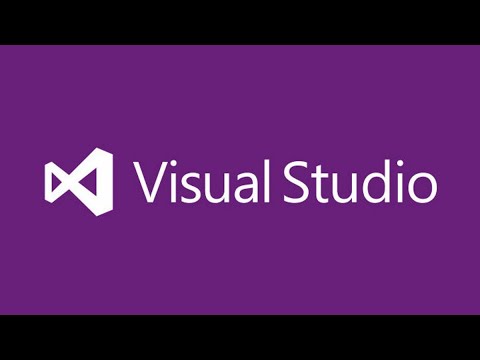This image features a minimalist design dominated by three primary colors. At the top and bottom of the image are two black rectangular bars, relatively thin but prominent against the background. Between these bars lies a plain, dark purple background. Centered on this purple expanse is the text "Visual Studio," with the 'V' and 'S' capitalized and the remaining letters in lowercase, formatted as "VisualStudio." Adjacent to the text is a logo depicting two overlapping triangles with a slight 3D effect. The left triangle is smaller, while the right triangle is larger, both meeting at their pointy ends to create a cohesive and modern visual impression.